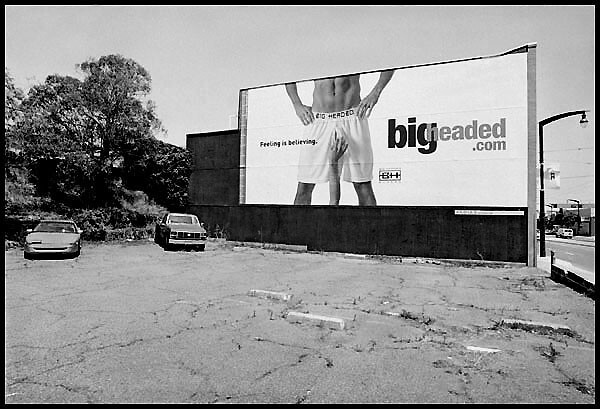The photograph depicts a weathered parking lot with cracked asphalt, some patches filled with tar, and occasional tufts of grass poking through. Two vehicles are noticeably backed into the lot—a spaced-out sedan and a pickup truck. Dominating the scene is a large, provocative billboard at the far end of the lot. The billboard is primarily white with stark black text, prominently featuring the website "bigheaded.com" and the phrase "Feeling is believing." At the center of the billboard stands a man showcasing his abs while clad in white boxer shorts emblazoned with the "bigheaded" logo. A hand reaches up from the bottom of the billboard, provocatively positioned near the man's groin area. To the right of the billboard, a solitary streetlight stands against the backdrop of a roadway. Encircling the scene on the left, deciduous trees with full foliage add a touch of nature to the otherwise urban tableau. The overall image is rendered in shades of black and gray, giving it a monochromatic, almost timeless feel.